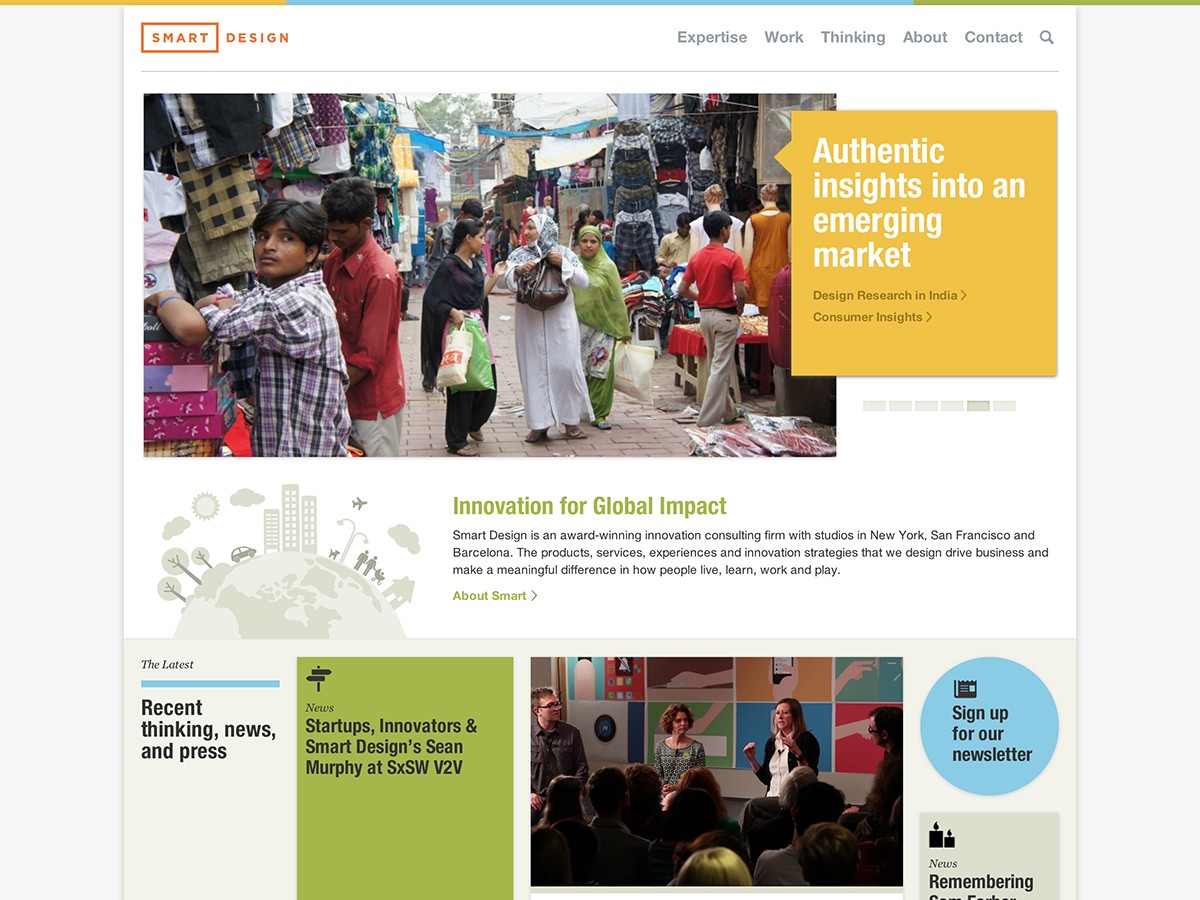A bustling street scene captures a vibrant marketplace in India, teeming with shoppers. Women, adorned in traditional long garments that flow down to their ankles, carry plastic shopping bags, while teenage boys navigate through the crowd. The atmosphere is lively, reflecting a typical day of commerce and social interaction. 

Adjacent to the image, text reads "Authentic insights into an emerging market," followed by promotional content for Design Research in India and Consumer Insights. It highlights "Innovation for global impact," shedding light on Smart Design, an award-winning innovation consulting firm with studios in New York, San Francisco, and Barcelona. The narrative emphasizes how the firm's designed products, services, experiences, and strategies drive business and significantly impact how people live, learn, work, and play. 

Additionally, there's a prompt to sign up for a newsletter. Another inset image features a woman delivering a speech to an attentive audience, further underscoring the firm’s commitment to innovation and impactful communication.